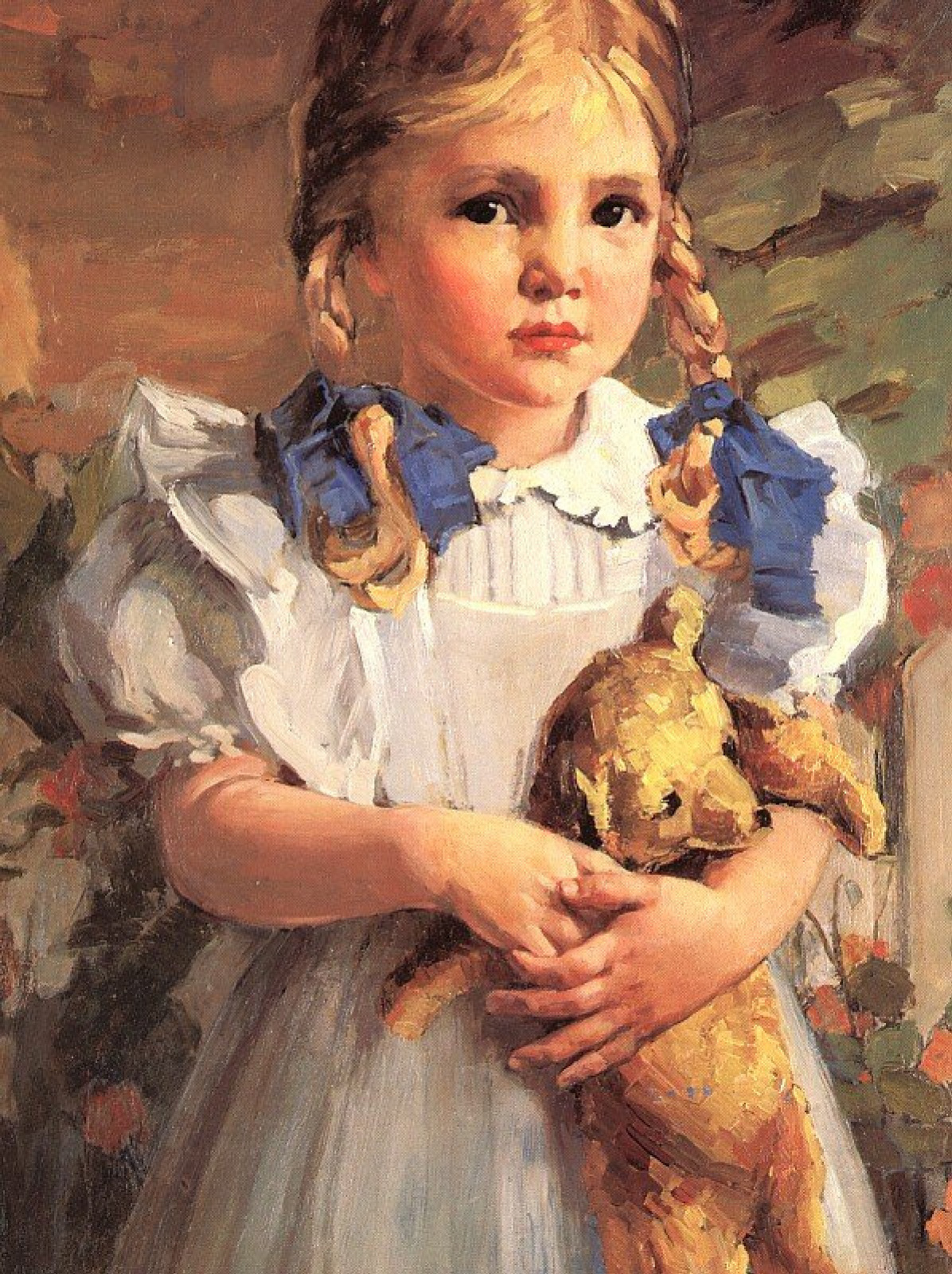The painting depicts a young Caucasian girl, approximately seven or eight years old, captured in a compelling close-up view. Her blonde hair is parted to the side, styled into pigtails that fall just below her collarbone, adorned with dark blue ribbons. She has large, expressive dark eyes that convey a sense of sadness, with her gaze seeming to look right through the viewer. Her delicate features include rosy cheeks, a small nose, and small red pouty lips. 

She is dressed in a light-colored dress, detailed with a white collar and puffy short sleeves that extend outward. The dress has a white apron overlay. Her arms are folded, clasping a brown teddy bear tightly against her chest, adding to the overall sense of melancholy. The background is abstract, painted with swatches of gray, red, and black, providing no distinct setting but focusing the viewer’s attention on the little girl and her poignant expression. The intimate composition of the image, with its close crop from her knees upwards and the partial cut-off at the top of her head, emphasizes the emotional depth captured by the painter.